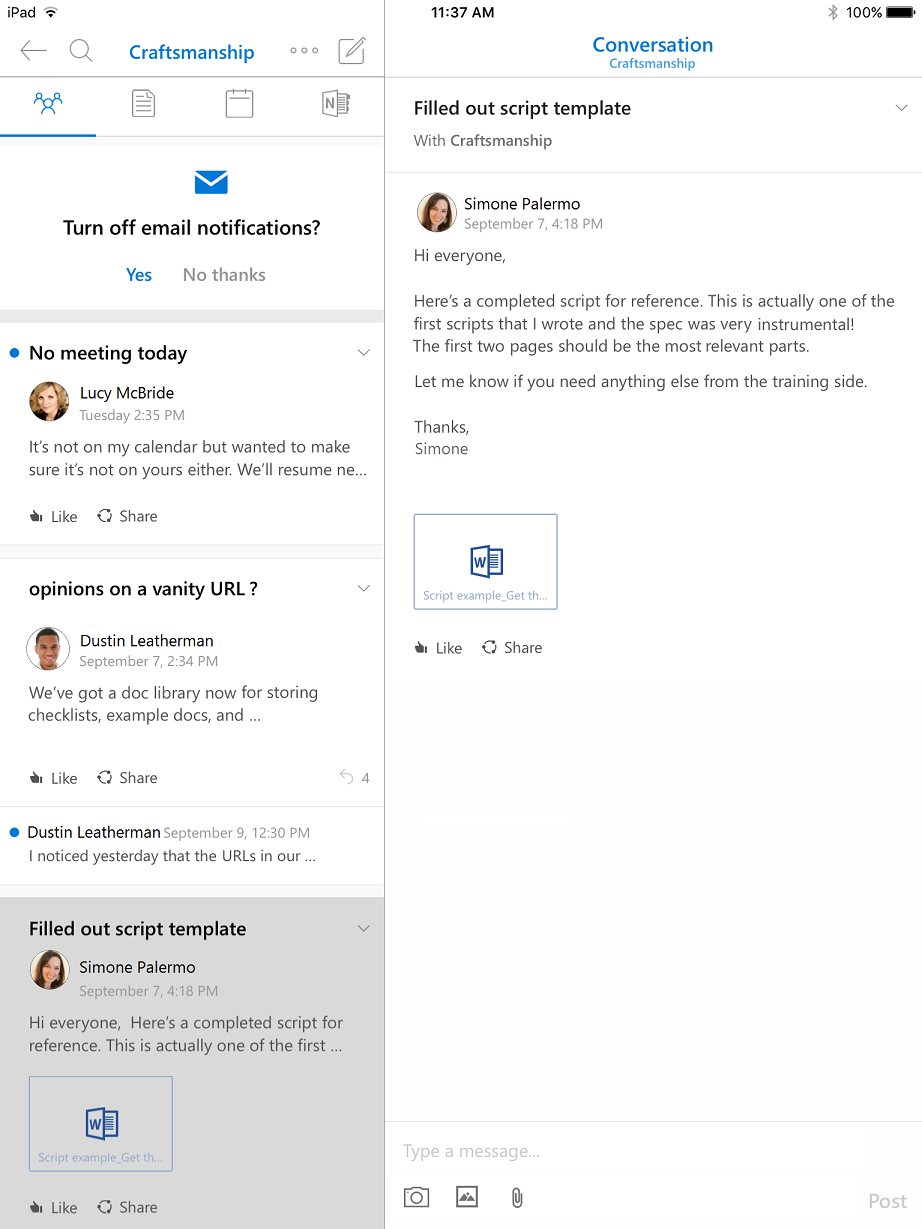A detailed descriptive caption for the given image could be:

The screenshot captures a digital interface with a predominantly white background. In the top right corner, the device shows a full battery icon with a 100% charge and a timestamp of 11:37 a.m. On the left-hand side, a vertical navigation menu is visible. The top label "Craftsmanship" is highlighted in blue. The menu includes a series of icons: one depicting three people (which is currently selected), a document icon, and a calendar icon. Below these icons, there is an option to "Turn off email notifications," with choices "Yes" and "No, thanks."

The main section of the screenshot features a feed with several posts. The top post, authored by Lucy McBride at 2:35 p.m. on a Tuesday, reads: "No meeting today. It's not on my calendar, but wanted to make sure it's not on yours either. We'll resume any..." The next post is by Dustin Leatherman, dated September 7th at 2:34 p.m., discussing opinions on a vanity URL with a message that starts, "We've got a doc library now for storing checklists, example docs, and..." A subsequent post by Dustin, dated September 9th at 12:30 p.m., mentions, "I noticed yesterday that the URL's in R..."

At the bottom is a gray input box, above which is a post by Simone Palermo, dated September 7th at 4:18 p.m., stating: "Hi, everyone, here's a completed script for reference. This is actually one of the first..." An attached Word document accompanies this message. On the right side of the screen, the content of this email is open, displaying the completed text: "Hi, everyone, here's a completed script for reference. This is actually one of the first scripts that I wrote, and the spec was very instrumental. The first two pages should be the most relevant parts. Let me know if you need anything else from the training side. Thanks, Simone."